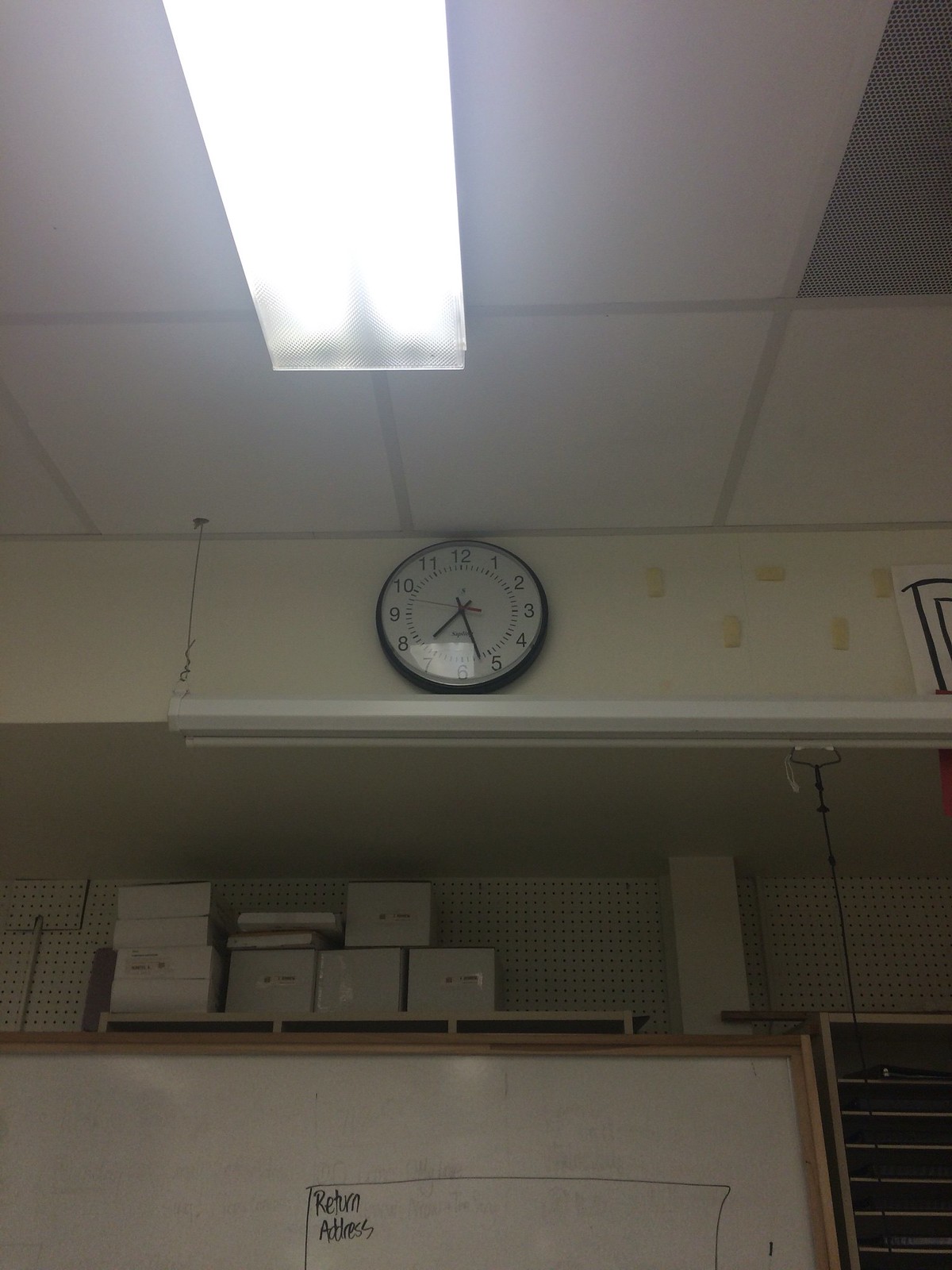The image depicts a classroom captured from a floor perspective, focused upward toward the ceiling. Prominently, there is a white clock with a black rim and large black hands, showing a time approaching 7:30, though it's uncertain if it's a.m. or p.m. The ceiling features large panels with a long, rectangular fluorescent light extending toward the upper left of the frame. Below the clock, there's a shelf holding some white boxes, and a pegboard backing it. Further down, a whiteboard with a drawn rectangle labeled "return address" in black ink is positioned. Adjacent to the whiteboard on the right side, there's a multi-layered shelf system likely used for sorting or storing papers. The image also shows remnants of tape on the wall, suggesting something has been recently removed.